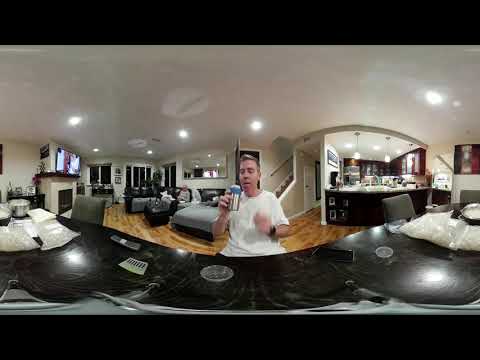In this detailed image, we see an older Caucasian gentleman with short blondish hair, sitting at what appears to be a large black countertop that could also be a dining room table in his home. He is wearing a white t-shirt and a watch on his left arm while holding a can, possibly a beer can, in his right hand. The setting seems to be indoors at night, giving a cozy atmosphere to the scene. 

The man's house has a modern design with beige walls and a wooden floor. To the man's left, we see a living room featuring a large couch and additional seating, and a TV mounted above a fireplace, which is currently turned on. The room is equipped with multiple built-in ceiling lights. 

On the right side of the image, there's a view of the kitchen, characterized by black cabinets and grayish-white countertops, with striking red walls. In the background, there is also a staircase and a hallway leading to other parts of the house. The image appears to be slightly distorted, likely due to a 360-degree panoramic view, enhancing the expansive feel of the home.